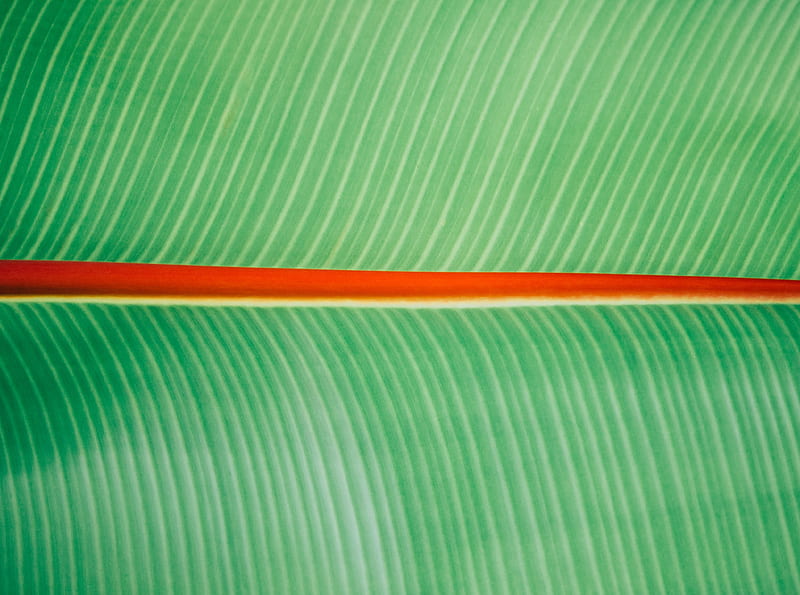The image showcases a highly detailed and zoomed-in view of what appears to be a leaf or possibly a painting inspired by a leaf's close-up. Central to the image is a thick horizontal red line, accentuated by a thinner white or yellow line beneath it. The background predominately features rich green hues, interspersed with lighter green or white vertical stripes, adding depth and texture. The composition gives an impression of a slight curve, with the top green section tilting to the right and the bottom section also moving right but at a different angle. The precise and vivid depiction, with the leaf extending horizontally across the image rather than vertically, lends to its almost perfect and artistic appearance.